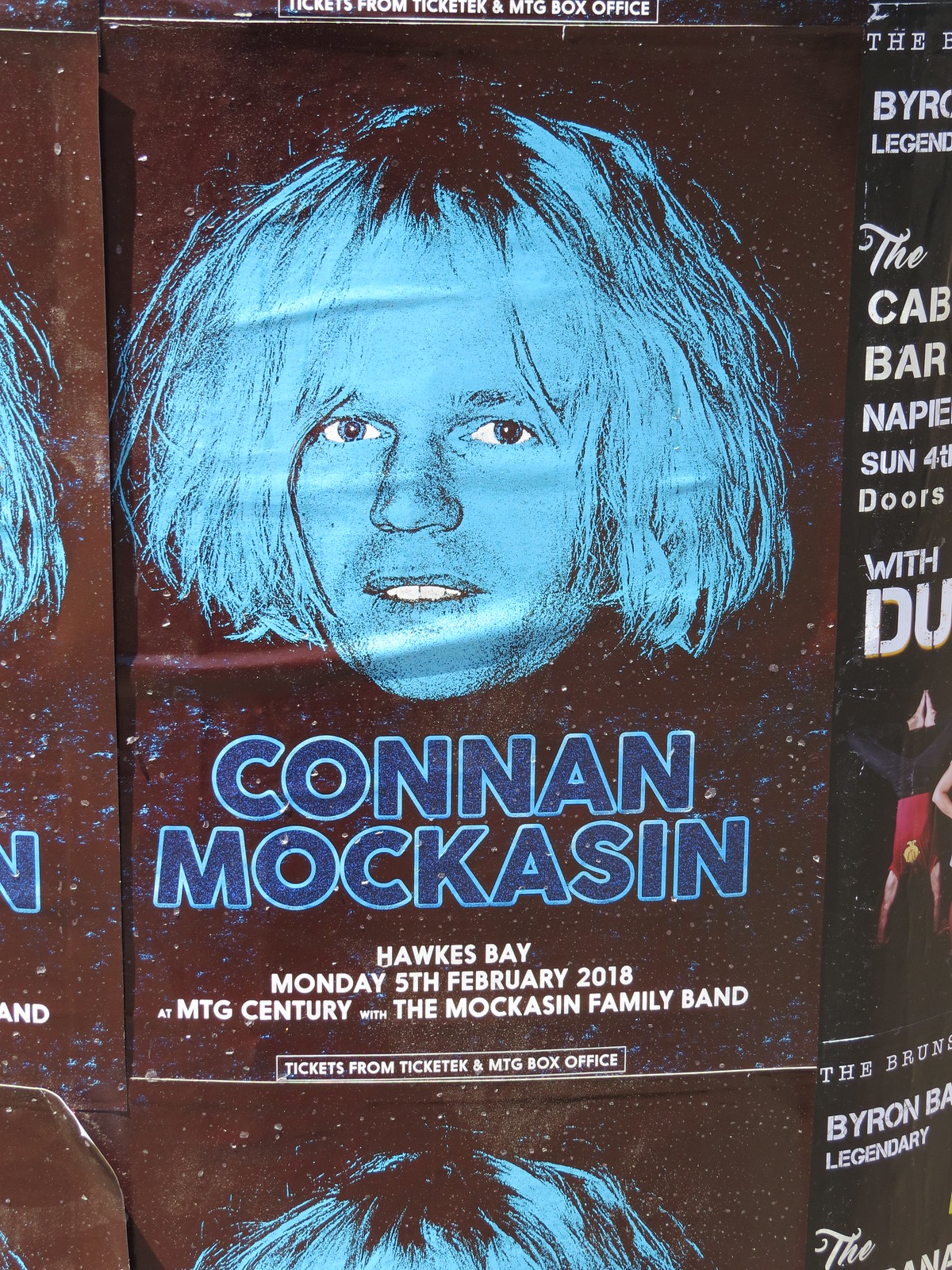A billboard sign hangs against a dark, star-dappled background, resembling a night sky. At the center is a pencil-drawn image of Conan Moccasin, his long, white-blond hair framing a face colored in a striking blue hue. His piercing blue eyes stand out, making a captivating focal point. The name "Conan Moccasin" appears below the image in dark blue, capital letters, outlined with light blue, giving it a glowing effect. Beneath the name, in smaller white text, it announces the event details: "Hawks Bay, Monday, February 5th, 2018 at MTG Century with the Moccasin Family Band." Additional information about tickets is provided in white letters within a white-outlined box on the right side, partially visible in the photo, stating "Tickets from Ticket Tech and MTG Box Office."